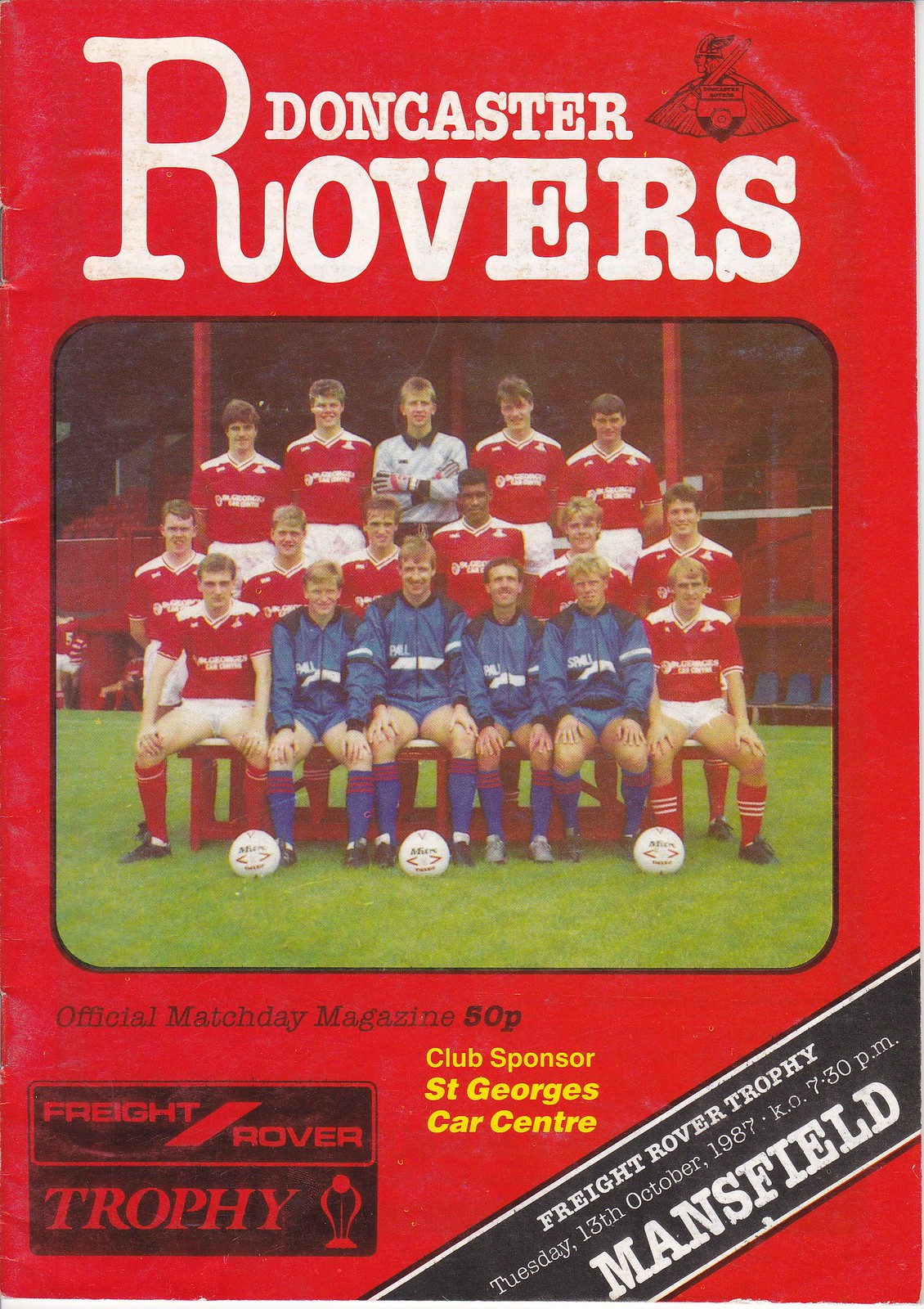This is the cover of an old football game day program, prominently featuring a bright red background. At the top, "Doncaster Rovers" is written in large white text. In the upper right-hand corner, there's a small black insignia depicting a Viking with a cape, sword, and shield. Below this, a central, bordered photograph shows the Doncaster Rovers soccer team arranged in three rows: the front row features four players in blue and white uniforms, while the rest of the team is in red and white, except for one player in the back row dressed in all white. Three soccer balls are positioned in front of them on green grass. Directly beneath this photograph, white text reads "Official Match Day Magazine 50p." Following this, in yellow text, is "Club Sponsor St. George's Car Center." On the bottom left, a black square indicates an advertisement for the "Freight Rover Trophy." A black diagonal banner extends from the bottom right corner to the center, with white text announcing "Freight Rover Trophy Tuesday 13th October 1987 kickoff 7:30 p.m. Mansfield."